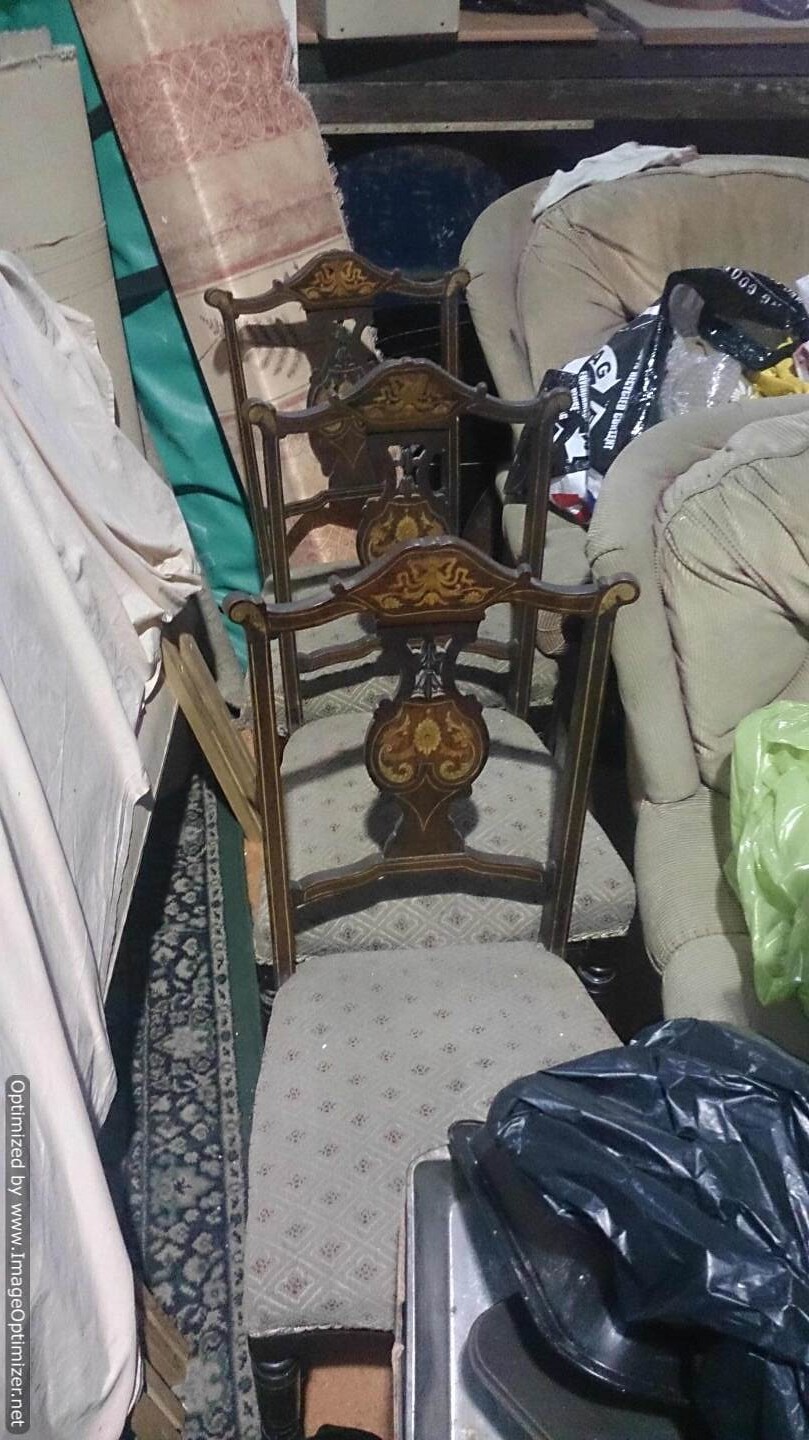The color photograph captures a crowded storage room filled with an assortment of furniture and items. In the center, three wooden dining room chairs are lined up, each featuring carved backs adorned with yellow painted designs and cushions adorned in gray or white embroidery. Beneath the chairs lies an ornate oriental rug showcasing blue and teal hues. To the right side of the image, partially visible beige sofas are buried under a mix of clear, black, and green plastic bags. In the foreground, a black garbage bag sits on a silver tray near the bottom right corner. Behind the chairs, a pink cloth with metallic embroidery is draped over objects, accompanied by a roll of beige carpet and what appears to be wallpaper or wrapping paper. In the left part of the image, a white sheet is draped over unidentified furniture. The entire room is densely packed, resembling an attic or a space where items have been haphazardly stored, creating an overall impression of clutter and congestion.